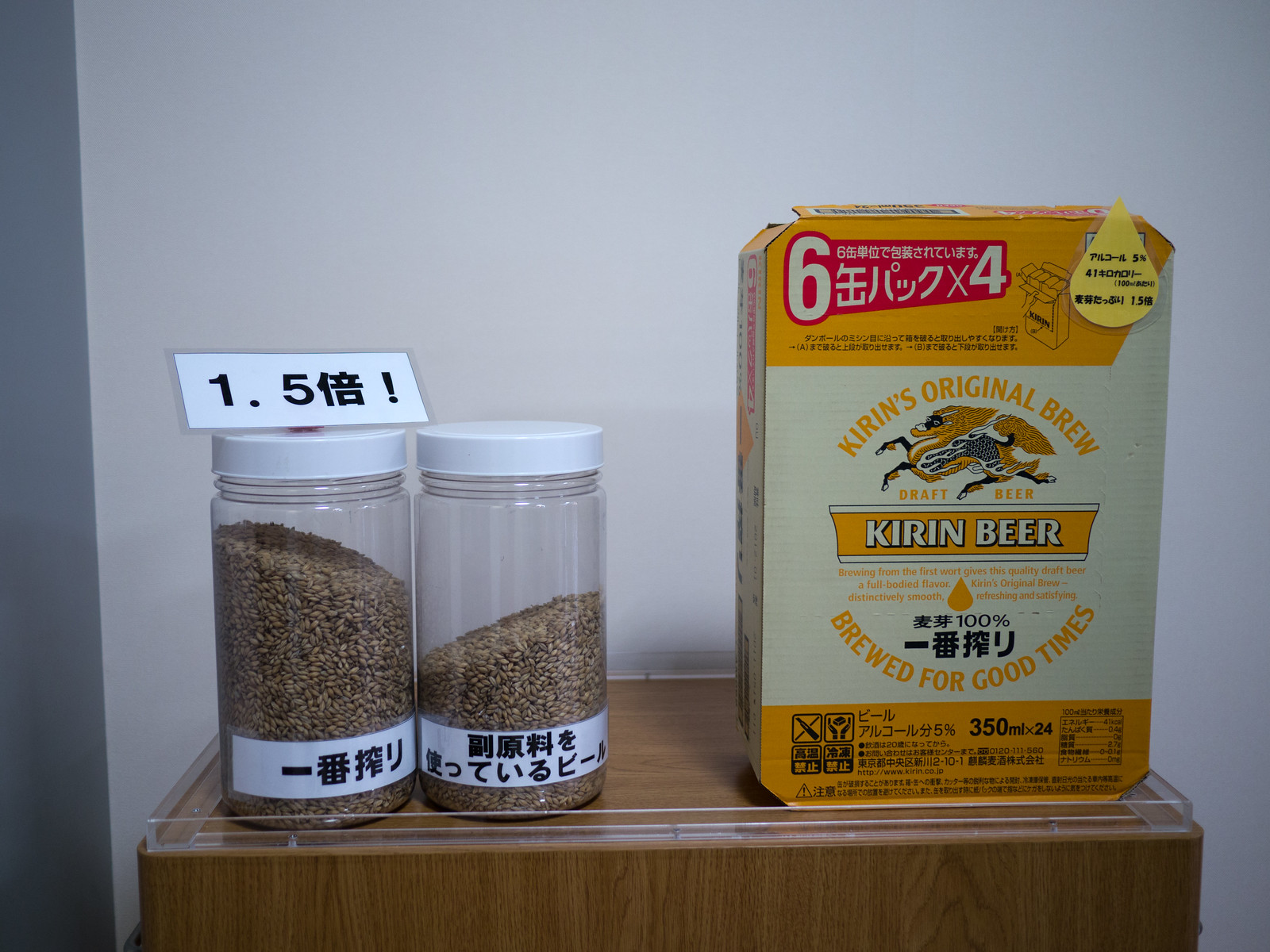A detailed image of a wooden table adorned with various items positioned against a white wall. On the left side of the table, there are two clear jars with white lids, containing barley or seeds. Each jar features a white label with black Chinese or Japanese symbols. The leftmost jar has a small sign on top, displaying "1.5" followed by an exclamation mark. To the right of these jars, there is a tan and yellow cardboard box with accents of red and black, labeled "Kieran Beer" and "Kieran's Original Brew". This box prominently displays the text "brewed for good times," and features a logo of a dragon-horse, with a teardrop-shaped yellow mark around it. The box also notes "Draft Beer" and has the measurements "350 milliliters by 24" printed on it. The items are placed on a wooden shelf that is topped with a clear plexiglass tray, adding to the overall neat and orderly presentation.